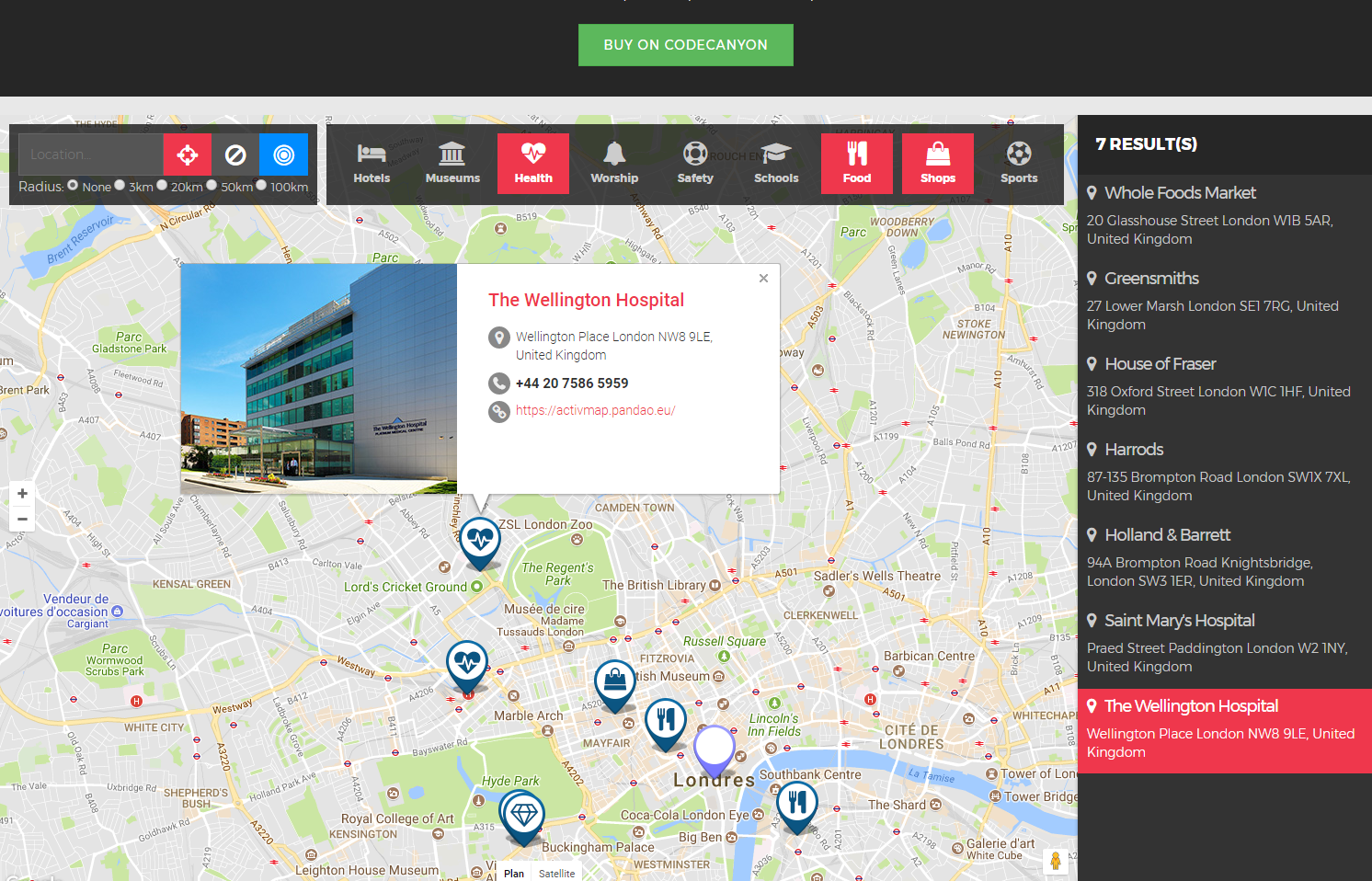Here's a cleaned-up and detailed caption for the image description:

---

This image is a screenshot of a computer screen predominantly displaying a digital map on the left side. The map features various tagged locations including restaurants, shopping centers, and hospitals. The central focus of the map is the Wellington Hospital, highlighted by an informational pop-up near the top of the screen. This pop-up includes a photograph of the hospital—a gray building with many windows—and detailed information beside it: "The Wellington Hospital, Wellington Place, London, United Kingdom," along with a phone number and a website address.

At the top of the screen, there's a black navigation bar. Centered in this bar is a green button labeled "Buy on Code Canyon." Another toolbar below this bar shows several categories, with "Health" highlighted in red, accompanied by an icon of a heart, and "Food" and "Shops" also selected. These selections correspond to the types of locations currently displayed on the map.

---